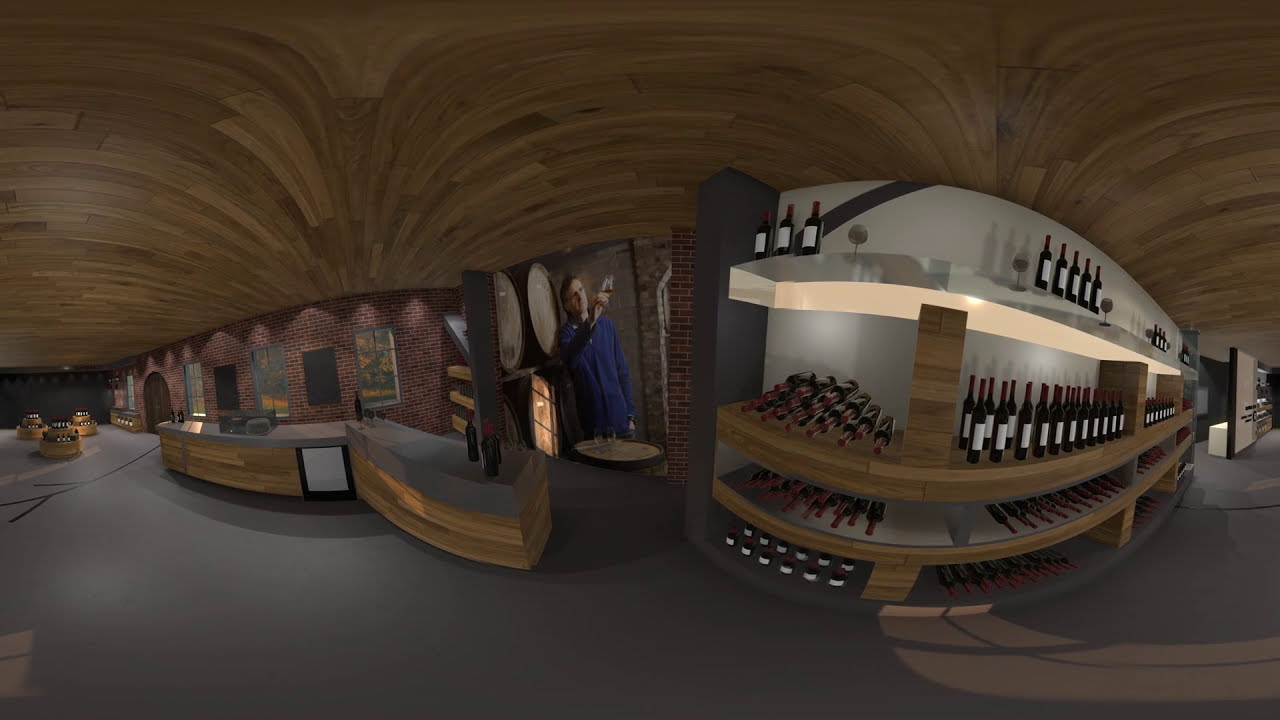The image depicts a computerized rendering of a cozy, indoor restaurant or liquor store. The space features a distinctive brown wooden ceiling and a plain gray cement floor. Along the right-hand side, four horizontal shelves are filled with uniform-looking wine bottles, some standing upright while others lie on their sides, with a few wine glasses interspersed. The storage area behind the counter showcases these bottles with white labels and red caps, under subtle shelf lighting. The setting also includes a brick wall and a counter area where customers would typically place orders or pay, though there are no customers present in the scene. Dominating the left side, a photograph of a Caucasian man in a long-sleeve blue button-down shirt is superimposed; he stands beside bourbon barrels, holding a glass of wine in his right hand. The atmosphere is dimly lit, with no prominent ceiling lighting or chandeliers, and additional paintings decorate the remaining walls.